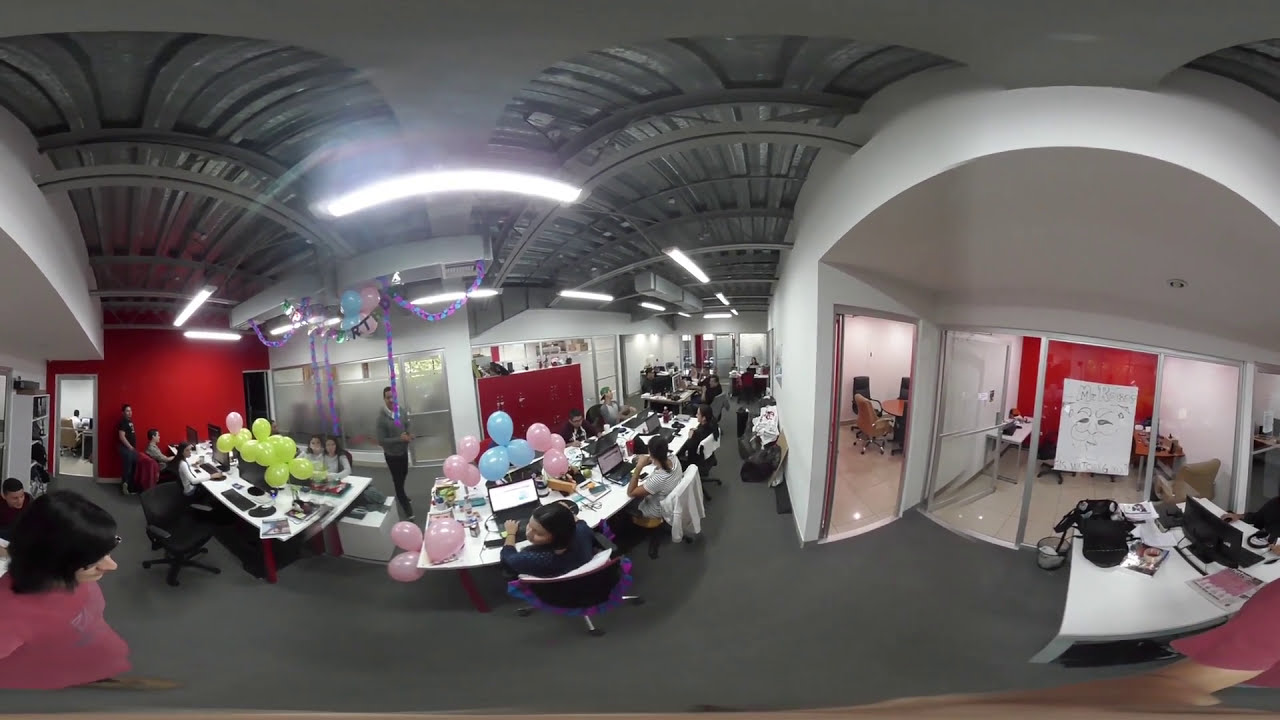This panoramic image captures an active corporate office space with a celebration taking place. The room features a distinctive white and red color scheme, with a red wall to the left and a white wall extending over a glass doorway. The floor is carpeted in gray, and people are seen working at curving, arch-shaped tables that dominate the space. Adding a festive touch, balloons of various colors—yellow, pink, and blue—are scattered on the tables and floor. The office is bustling with activity; several individuals are busy at their computers, while others are walking around. One woman in a pink shirt is particularly noticeable on the left-hand side, though there is some visual distortion near her. The background showcases a metallic, open-ceiling design featuring arch shapes and fluorescent lights, further emphasizing the modern and energetic atmosphere. Glass doors on the right lead into another room, reinforcing the open-plan design of this vibrant workspace.